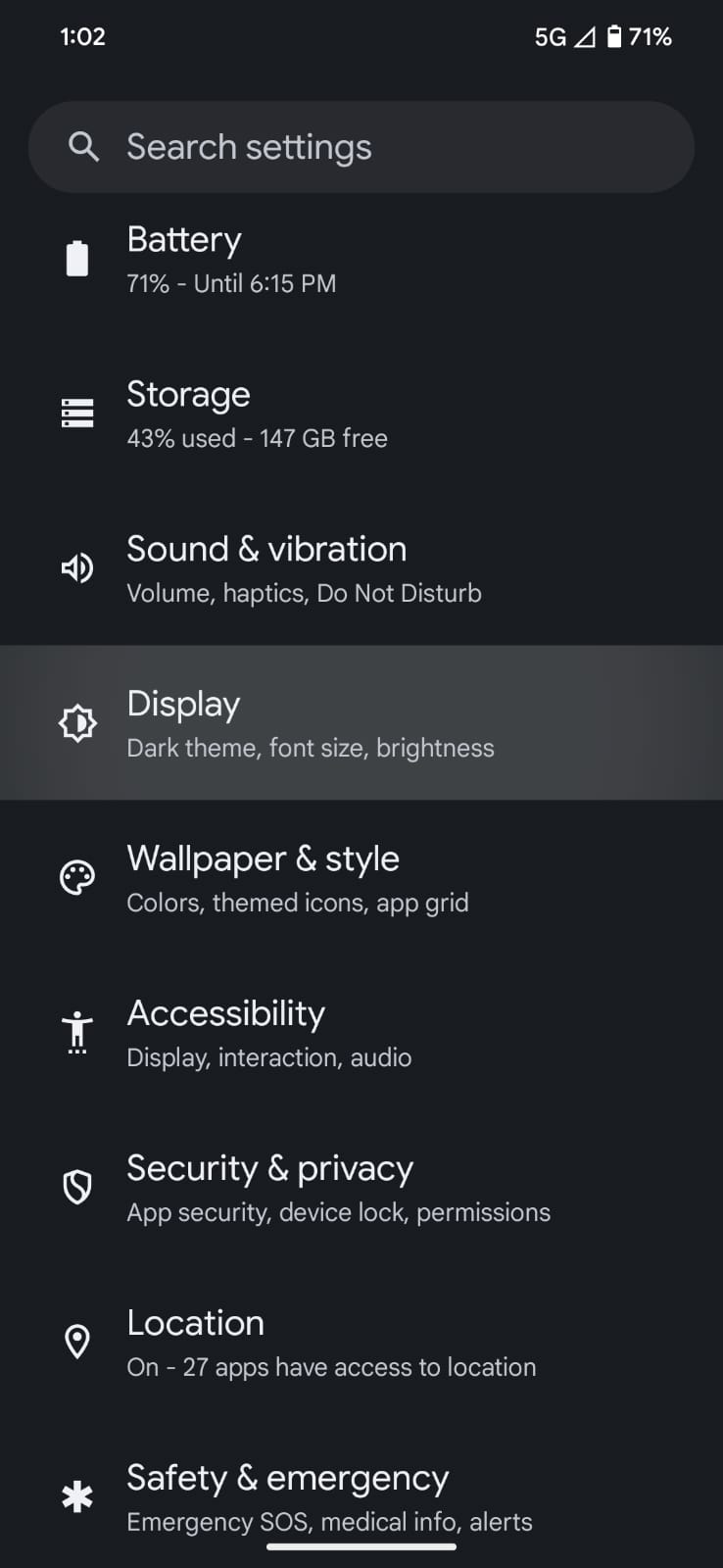Detailed Caption: 

The image displays a smartphone screen that is currently active, showcasing various settings and information at a glance. At the top left corner of the screen, the status bar indicates "5G" connectivity and the time "1:02 PM." The battery icon is visible with a charge level of "71%" and an estimated duration until "6:15 PM." 

Below the status bar, there is a "Search" option and access to "Settings." The screen shows detailed device statistics including "Storage" usage at "43%" with "47GB free." Additionally, it mentions sound settings such as "Sound and Vibration," "Volume," and "Haptics." The "Do Not Disturb" mode is also highlighted.

The display settings include "Dark Theme," "Font Size," and "Brightness." There is an option for "Wallpaper and Style," which includes "Colors" and "Themed Icons," as well as the "App Grid."

In the "Accessibility" section, the screen features settings for "Display," "Interaction," and "Audio." It also covers "Security and Privacy," mentioning "App Security," "Device Lock," and "Permissions." Location services are "ON," with "27 apps" having access to location data.

In the "Safety and Emergency" section, the screen includes features like "Emergency SOS" and "Medical Info Alerts."

The overall background of the screen is black with white text. There's a thin white line running horizontally across the bottom and the center, dividing sections or indicating a scroll bar for further options not currently visible in this image.